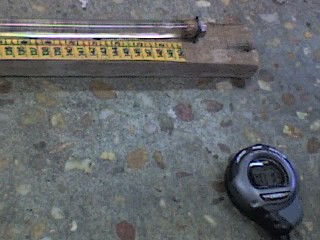This photograph features a wooden outdoor thermometer with a yellow stripe running vertically along its side, displaying temperature readings. The thermometer is positioned horizontally atop a terrazzo surface, characterized by a blend of gray concrete interspersed with white, brown, and dark brown pebbles. Placed below the thermometer is a small, round device resembling a countdown timer. This black timer has a digital readout encased in a bulbous plastic cover and includes a front button, likely used to start the timer.